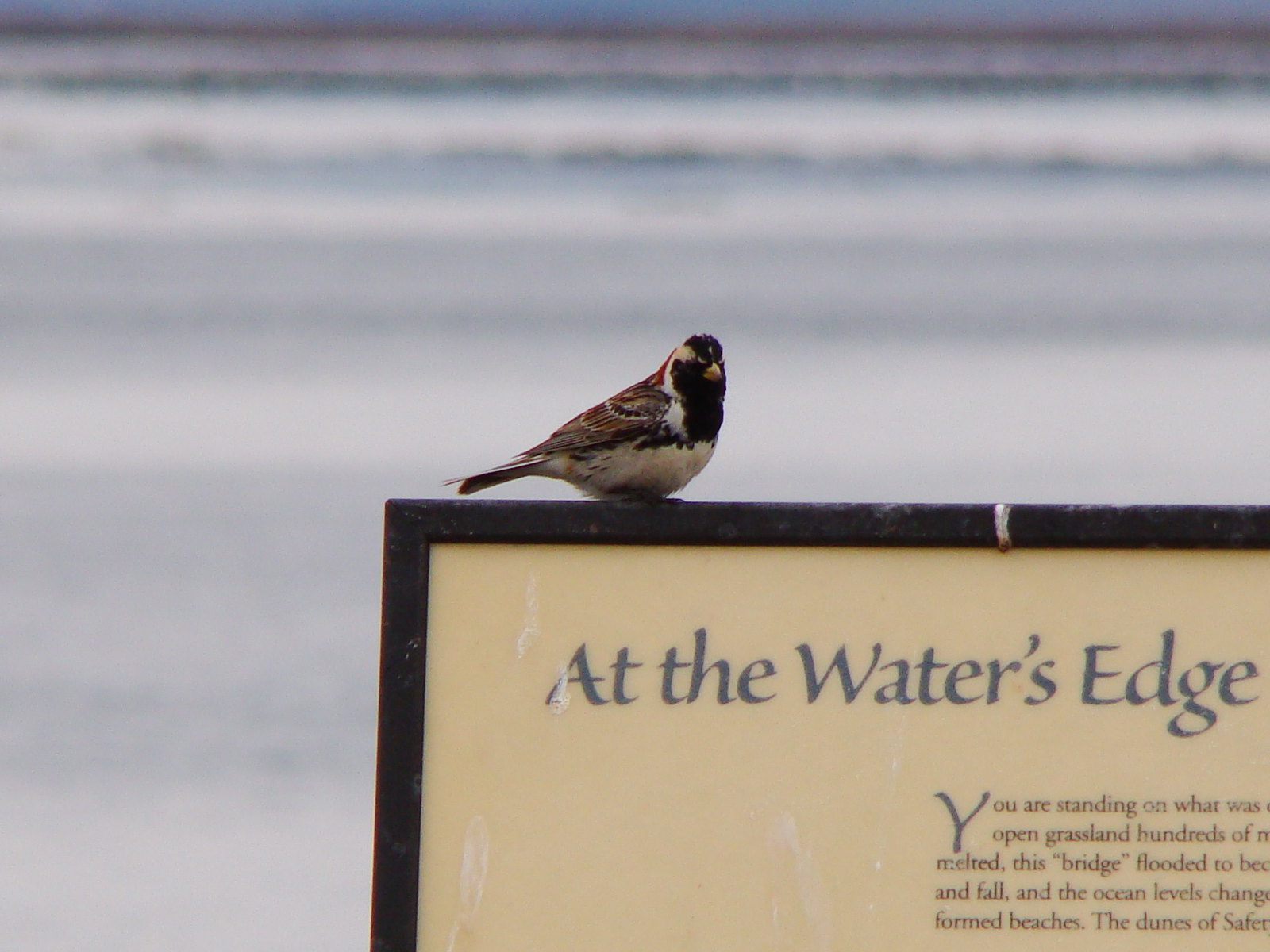The photograph captures a small bird perched on a framed plaque against a vast, blurry background of what appears to be a grayish-blue ocean or sea. The bird, centrally located and facing right, features a white belly, a yellow beak, and a black head with white markings. It also has a black breast, brown feathers on its back, some white around the eyes and down the neck, and a strip of red on its back. The plaque, occupying the bottom right side of the image, has a black border and a yellow background with blue text. The prominent title reads "At the water's edge," while the rest of the text, partially cropped out, starts with "you are standing on what was open grassland" and continues with fragmented phrases about melted bridges, flooded areas, ocean level changes, and the dunes of a place referred to as "Safe." The overall scene appears to be an outdoor setting, likely in a park near a body of water.